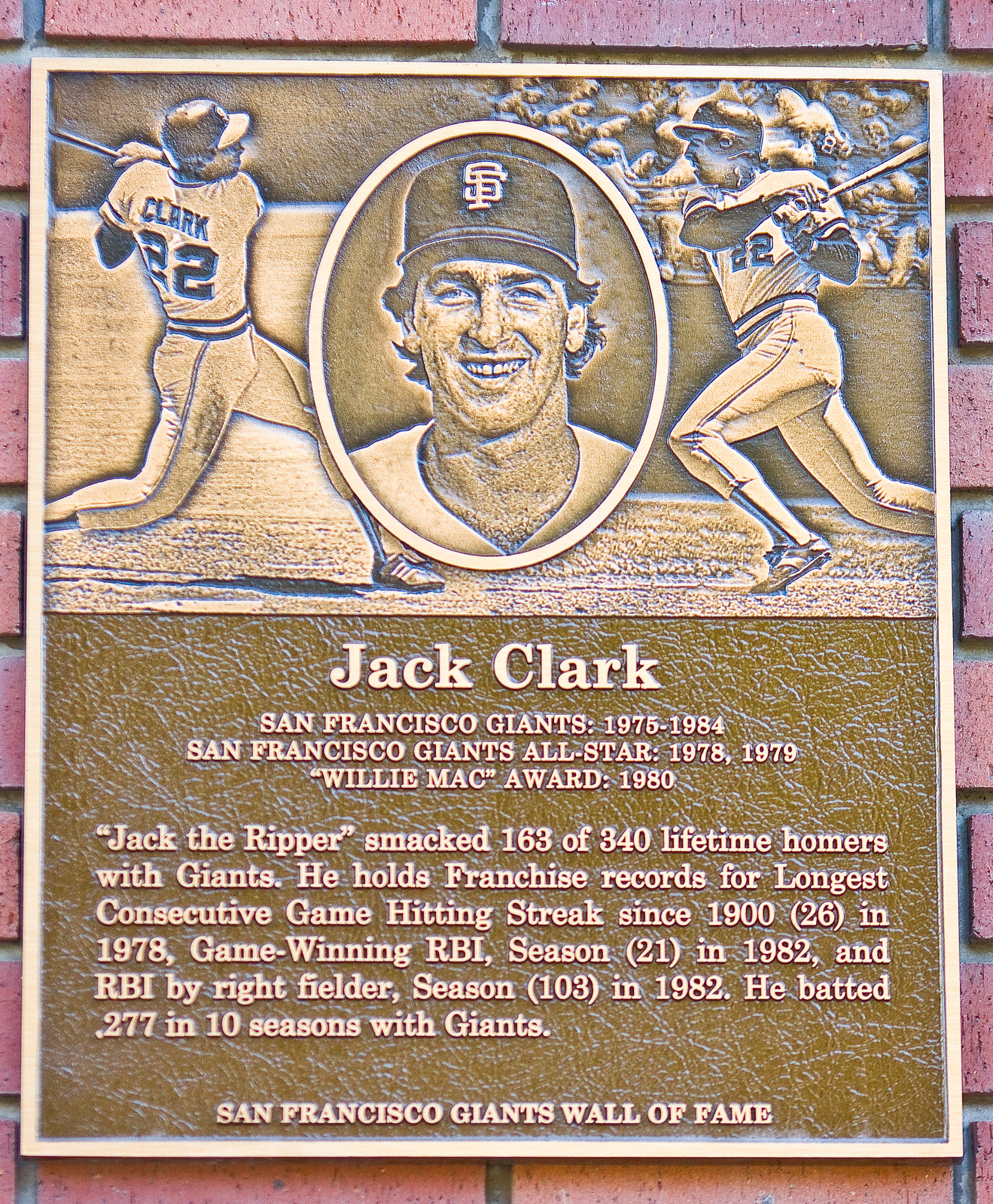The image depicts a bronze sports plaque affixed to a red brick wall, commemorating baseball player Jack Clark. The plaque, which has a light-colored border and a central bronze section, features etched images of Clark in various baseball poses. On the left side, Clark is shown from the back, preparing to swing a bat, while the right side presents a front-facing view of him in mid-swing. In the center, there's an oval portrait of Clark, showcasing his face with a baseball cap emblazoned with "SF," a toothy smile, thick eyebrows, and medium brown hair. Above the images, the plaque reads "Jack Clark, San Francisco Giants 1975-1984."

The text below the visuals honors Clark's achievements: "San Francisco Giants All-Star 1978-1979, Willie Mack Award 1980. 'Jack the Ripper' smacked 163 of his 340 lifetime homers with the Giants. He holds franchise records for the longest consecutive game-hitting streak (26) set in 1978, game-winning RBIs in a season (21) in 1982, and RBIs by a right fielder in a season (103) in 1982. He batted .277 over 10 seasons with the Giants." At the bottom, it notes, "San Francisco Giants Wall of Fame," further solidifying Jack Clark's legacy within the franchise.